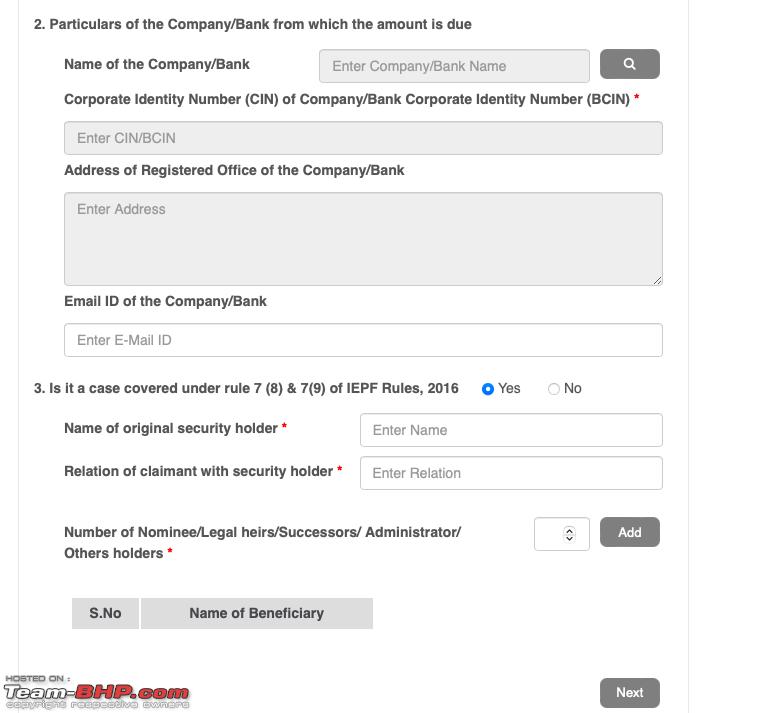This image depicts a form page with various fields for input. At the top of the page, there is a section titled, "Particulars of the Company/Bank from which the Amount is Due." This section contains the following fields:

1. **Name of the Company/Bank:** An open text box for entering the name.
2. **Corporate Identity Number of Company/Bank (BCIN):** A text box is provided to input the BCIN.
3. **Address of Registered Office of the Company/Bank:** A text field designated for the company's registered office address.
4. **E-mail ID of the Company/Bank:** A field to enter the email address.

Following these fields, there is a question regarding the case status under Rule 7, 8, and 9 of the IEPF Rules 2016, with a "Yes" and "No" option. The "Yes" option is selected and indicated with a blue marker.

Further down, the form asks for:

1. **Name of Original Security Holder**
2. **Relation of Claimant with the Security Holder**
3. **Number of Nominees/Legal Heirs/Successors/Administrators/Other Holders:** There is a blank box for entering this information.

At the bottom of the form, there is a section titled, "S.No, Name of Beneficiary."

In the corner of the page, the text "hosted on teambhp.com" is visible, and there is a gray "Next" button at the bottom.